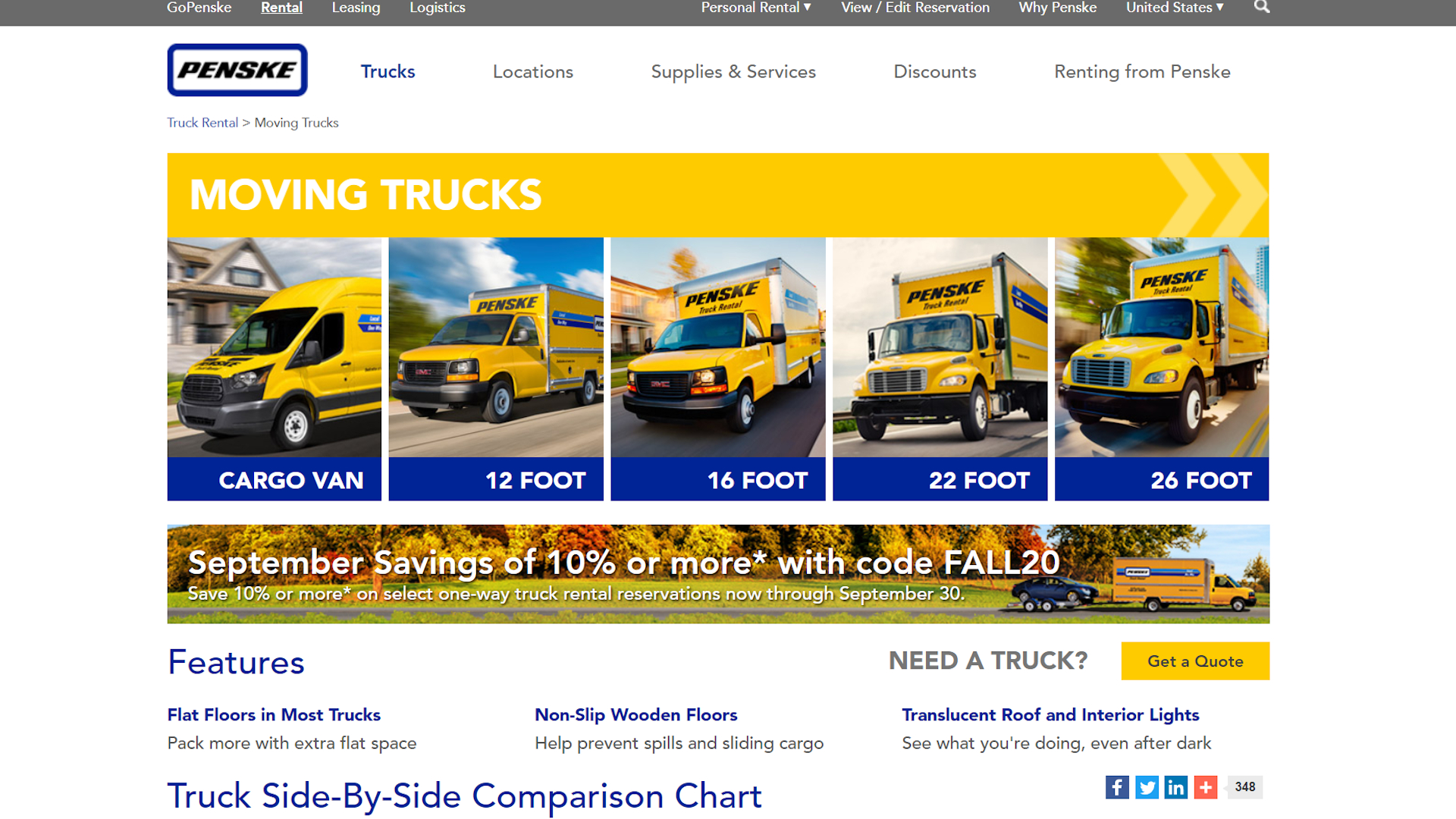The image showcases a web page for Penske Truck Rental. In the top left corner, the "Penske" logo, featuring black text with a blue border, is prominently displayed. Surrounding the logo at the very top of the page along a grey panel are selectable menu options, including "Go Penske," "Rental," "Leasing," "Logistics," "Personal Rental," "View/Edit Reservation," "Why Penske," and options for choosing the United States as the region and a search function.

Below the grey panel lies a white panel repeating the "Penske" logo and including additional navigation options like "Trucks," "Locations," "Supplies and Services," "Discounts," and "Rent from Penske." The "Trucks" option is currently selected, revealing various truck options.

A series of illustrative images of trucks is listed under "Trucks," showcasing different sizes: a cargo van, a 12-foot van, a 16-foot van, a 22-foot van, and a 26-foot van. All trucks are painted yellow with the Penske logo prominently displayed on the front.

Beneath these images, a separate panel advertises "September Savings" of 10% or more with the promo code "Fall20" and features a small picture of a car being towed by a rental truck.

Further down, the page includes general information on the features of the trucks, such as availability of flat floors in most trucks, non-slip wooden floors, translucent roofs, and interior lights. Users can conduct a side-by-side comparison of different trucks to determine the best option for their needs.